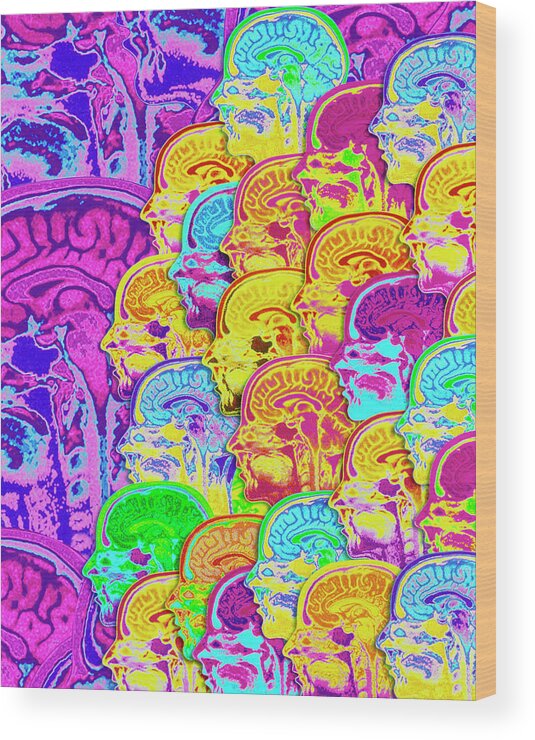The image is a computer-generated, poster-like artwork mounted on a wooden board. It measures roughly two feet by four feet and features a series of colorful, psychedelic human heads layered in rows and columns, each showcasing a detailed cross-section view of the brain and parts of the facial anatomy. The heads, likely from the same profile but depicted in various colors such as turquoise, pink, yellow, green, magenta, and blue, create a striking visual effect. The bottom row begins with four heads, progressively increasing in number to a total of six heads at the top. The colors are bright and highly saturated, adding to the psychedelic theme.

The right side of the image reveals the edge of the wooden board against a white background, while the brightly colored heads occupy about two-thirds of the artwork. The left side features a larger, abstract illustration of a head in purples, blues, and pinkish hues that the smaller profiles appear to be oriented toward, as if they are looking at this prominent figure. The outer edges of the picture emphasize the brains, especially in a prominent purple color, enhancing the surreal, vivid nature of the art.